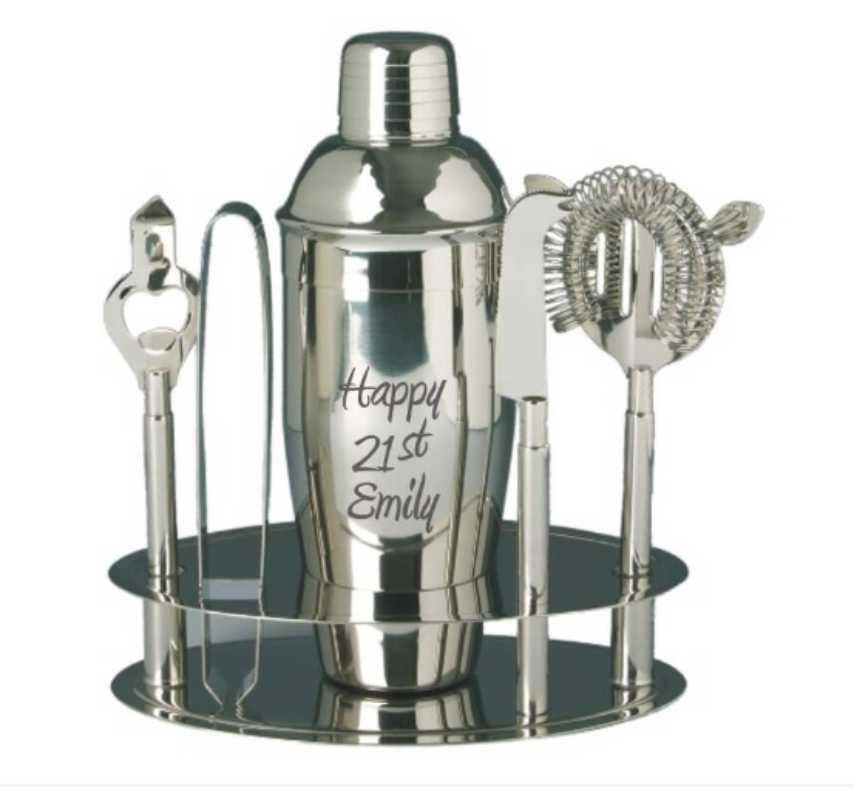This image features a polished silver cocktail shaker, prominently engraved with "Happy 21st, Emily." The shaker is reflective, with dark black reflections visible along its upper and lower parts. Surrounding the shaker are various bar tools neatly placed in a stand, which features two circular pieces: an upper one securing the tools and a lower one for their placement.

To the right of the shaker sits a strainer for ice, along with another chrome tool with springs. To the left, there's an ice tong followed by a chrome bottle opener and a notched knife. The cocktail set, with its elegant chrome finish, is not only practical but also a stylish celebratory keepsake.